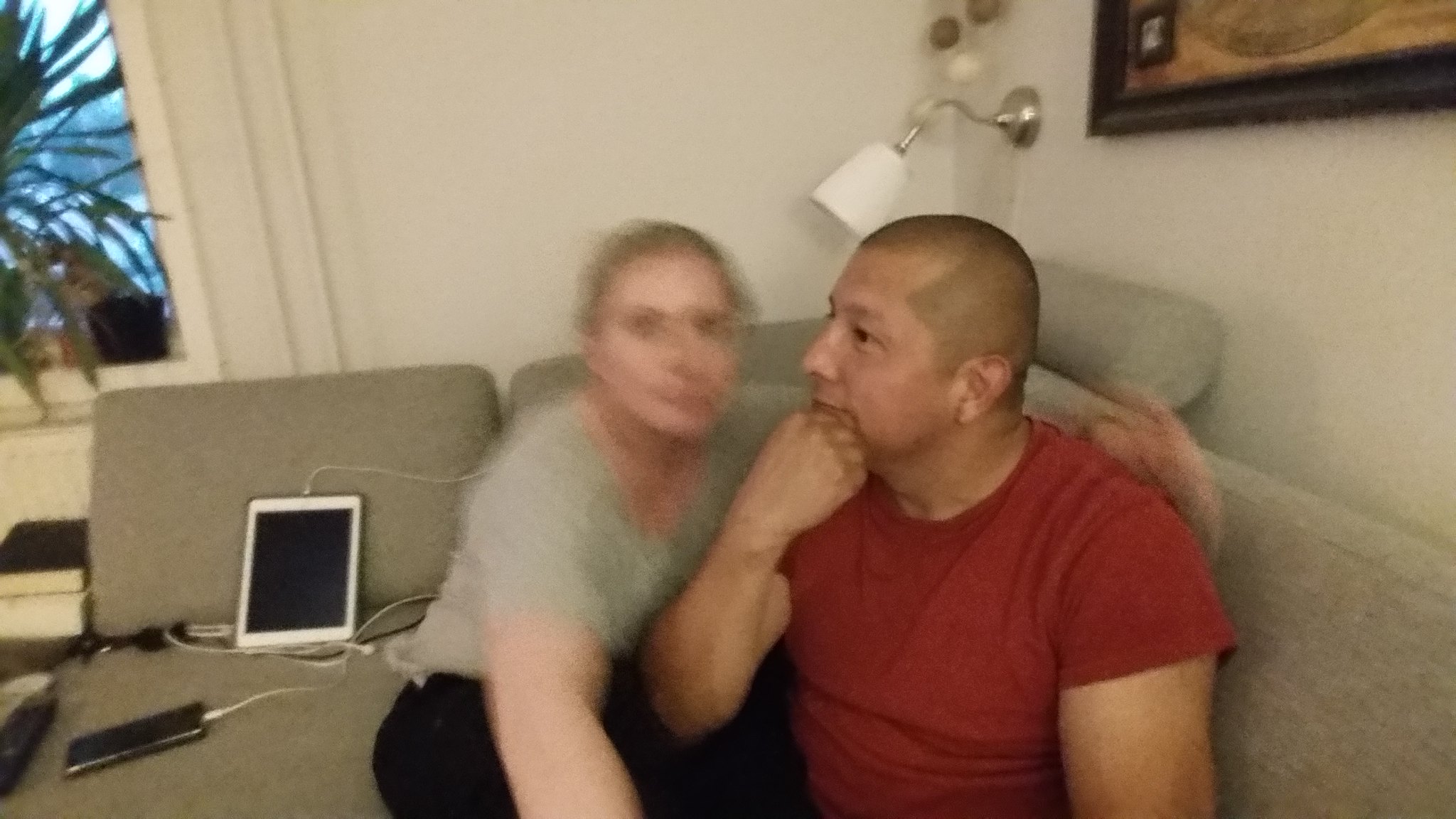In this image, two people are seated on a sofa. The person on the right is clearly visible and is decidedly male. He has a shaved head and is dressed in a red t-shirt. His head is resting on his fist, giving him a contemplative appearance. The individual on the left is more indistinct, especially in the facial area, making it difficult to determine their gender. They are wearing a grey t-shirt and appear to have their left arm draped around the person in red. Additionally, several electronic devices, including an iPad and a smartphone, can be seen charging nearby.